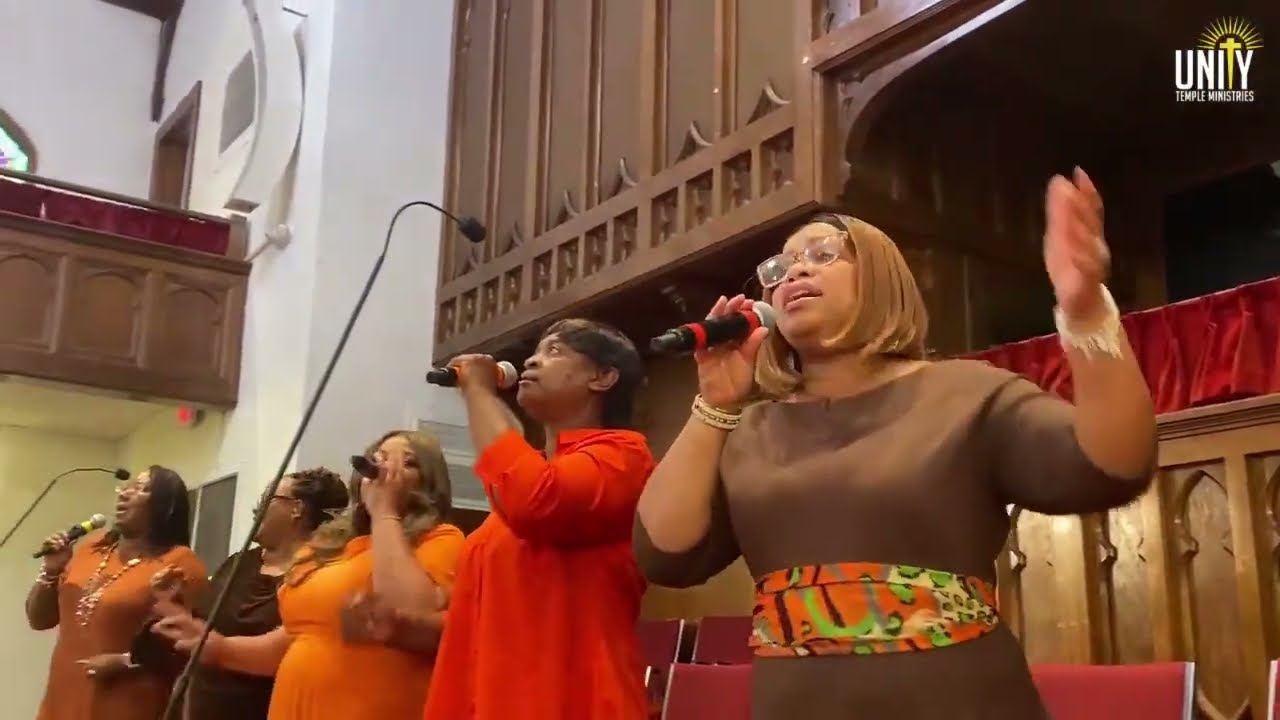This image captures five African-American women standing on a church stage, likely during a gospel performance at Unity Temple Ministries. Each woman is holding a microphone, and two additional stand microphones are positioned centrally. They are dressed in various shades of orange and brown: the woman on the far left wears glasses and an orangish-brown dress adorned with multiple necklaces and bracelets; next to her, a woman in a brown dress showcases a colorful belt around her waist; the center woman wears a vibrant orange dress; the next in line dons a reddish-orange dress; and the woman on the far right, who also sports glasses and has short blonde hair, is dressed in a medium-brown dress with a colorful belt. The backdrop includes wooden structures, white walls, a balcony, a stained glass window, and multiple red chairs. The upper right corner features the text "Unity Temple Ministries," with a distinctive yellow and golden cross forming the "T" in "Unity." The image appears to be a candid snapshot rather than a professional photograph. The overall color palette of the scene includes maroon, various shades of red and orange, blue, black, white, and numerous browns.